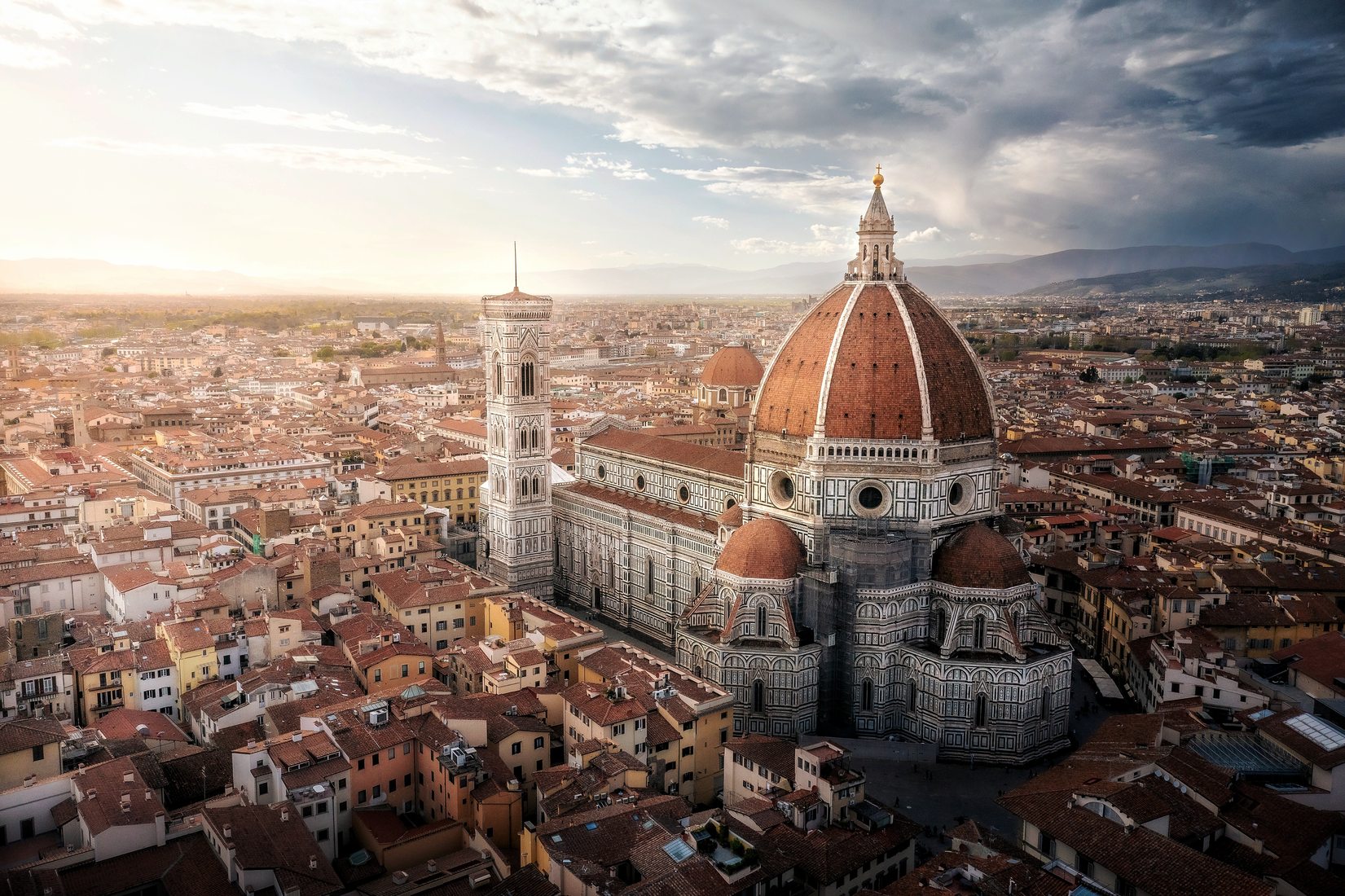This image captures an aerial view of Florence, Italy, dominated by a striking architectural centerpiece—a large building with a white and red exterior, featuring a prominent dome and smaller domes surrounding it, likely a significant church or historic building. The dome, with its weather vane on top, has distinct sections each adorned with nine small holes. Surrounding this central structure is a densely packed cityscape with a mix of buildings ranging from one to three stories high, predominantly residential rather than commercial.

In the background, a hazy silhouette of a mountain range stretches across the horizon, with the elevation rising higher towards the right edge of the image. The sky is mostly covered with large clouds, particularly concentrated on the right, but patches of blue sky are still visible, adding to the picturesque and somewhat moody atmosphere of the scene. This lack of greenery and open spaces highlights the crowded and bustling nature of this European cityscape.